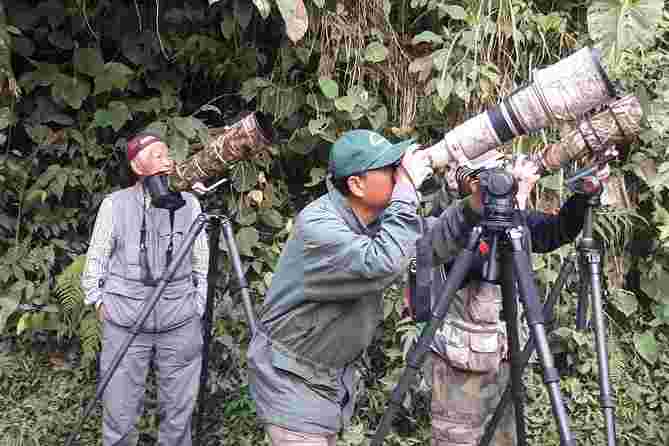The image depicts three older Asian men in a dense, lush green forest, possibly tropical or jungle-like, with thick foliage including palm fronds and large leaves, shaded in relative darkness but under an overcast yet bright daytime sky. Each man is positioned by a large tripod-mounted camouflage telescope. The man on the left, dressed in a gray jumpsuit and a red backwards baseball cap, is standing with his hands in his pockets, looking to his right as if taking a break. In the center foreground, another man is fully engaged with his telescope, wearing a greenish-gray jacket and a forward-facing green baseball cap, his face pressed to the lens looking upwards and to the right. Behind him, barely visible due to being partially obscured by the middle man's tripod, is a third individual in camouflage attire, similarly positioned with a telescope. The scene suggests they are on a nature observation expedition, possibly bird watching or observing wildlife high in the trees.